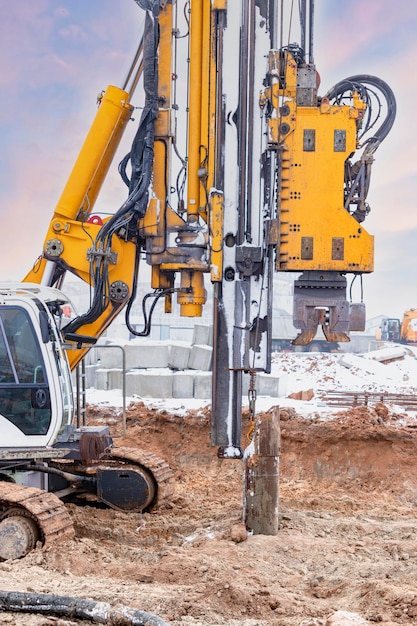This detailed color photograph, oriented in portrait, depicts a busy construction zone. Dominating the lower left of the image is a large bulldozer with a white operator cab. Attached to this machine is a long, bright yellow mechanical arm, featuring silver and black wiring. This arm serves as a heavy-duty drill used for penetrating the ground, likely to prepare for the installation of support pillars. The drilling tool is engaged in boring into a dirt surface, revealing a rusty brown round pipe at its base.

Surrounding this centerpiece are several notable elements: behind the bulldozer and drill, neatly stacked concrete blocks rest atop a snow-dusted ground, indicating recent snowfall. These blocks, along with other scattered construction materials and additional pieces of machinery, frame the midsection of the scene. The sky above is a cloudy purplish-pink, creating a stark contrast to the earth-toned hues below. Notably, the photograph focuses more on the heavy machinery and does not include visible workers, suggesting that the equipment may be operated remotely or the workers are out of the frame. The overall composition and realistic representation provide an in-depth view of the ongoing construction activities.